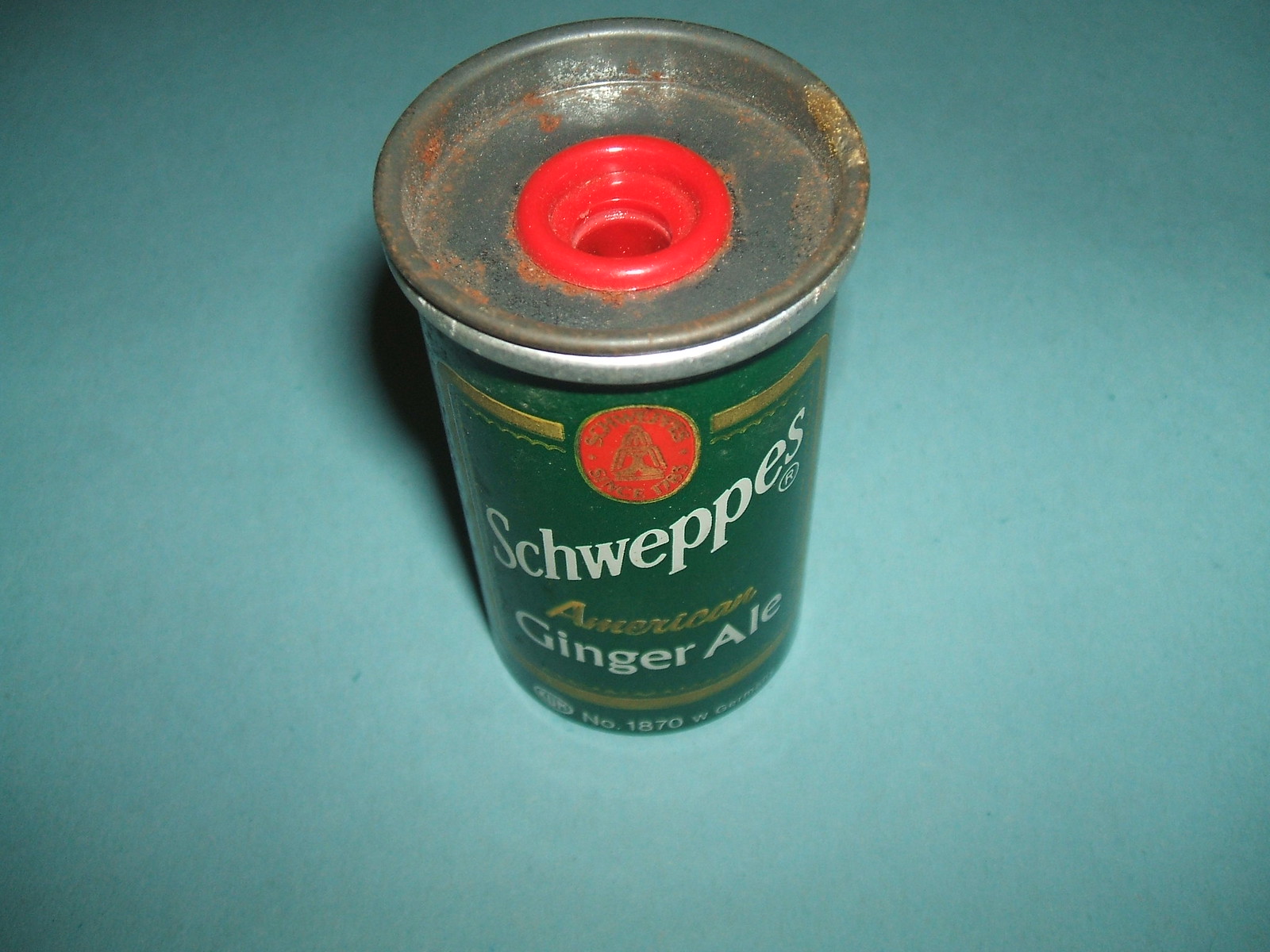In this horizontally oriented photograph, the focal point is a heavily rusted can of Schweppes Ginger Ale, prominently positioned at the center. The can's sides are a classic green, and it features a red medallion near the upper center with visible corrosion. Despite the rust, the branding is decipherable: "Schweppes" is written across the top, "Ginger Ale" in white print, and the word "American" nestled in gold between "Schweppes" and "Ginger Ale." At the bottom of the can, the inscription reads "NO 1870." The top of the can appears particularly weathered, showcasing deep rust with mottled patches of yellow and orange. Interestingly, this can has been modified with an inserted top and a conspicuous bright red inner plug that seems out of place yet fits snugly. The background is a gentle light green, providing a subtle contrast to the vibrant yet dilapidated can.